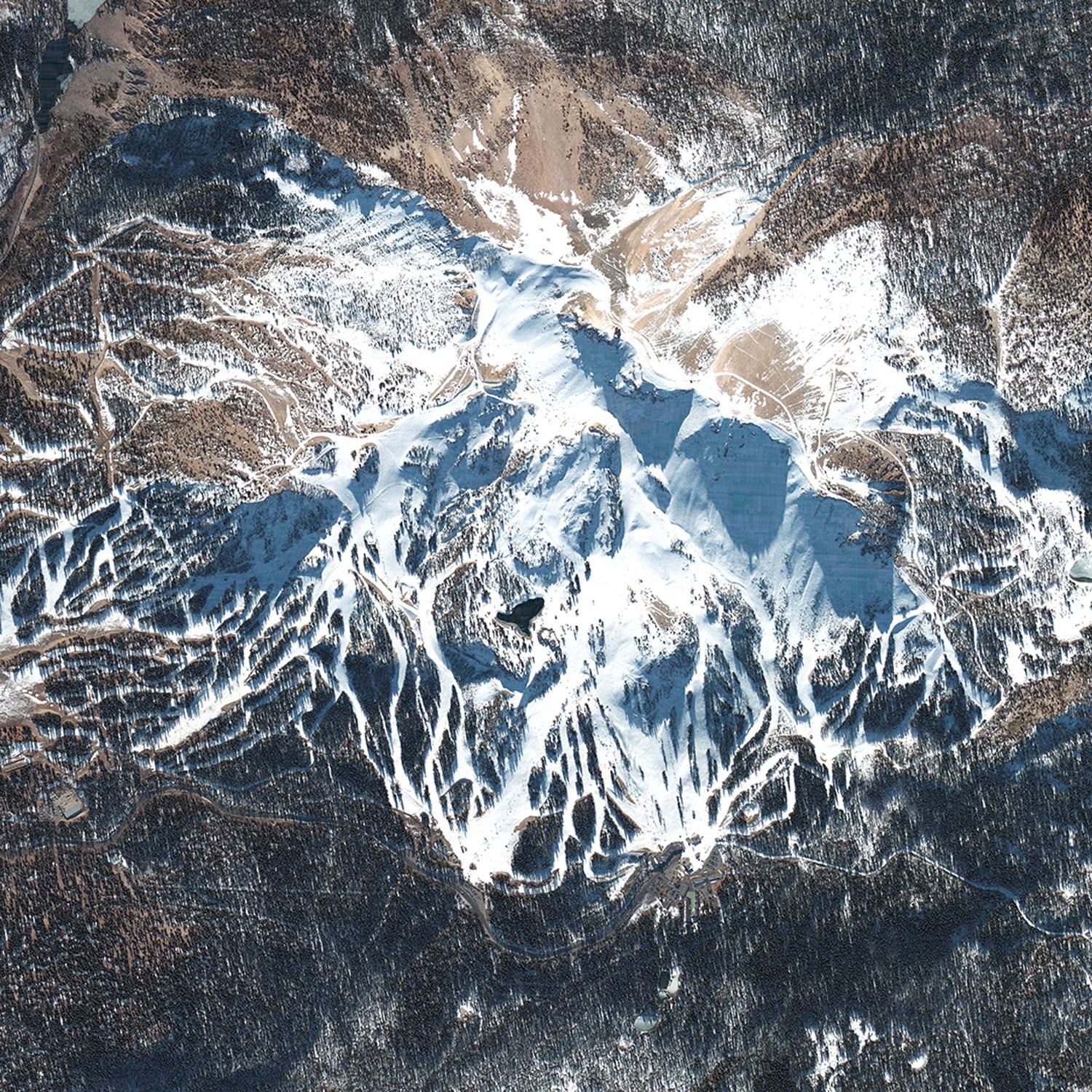This detailed aerial photograph, likely taken from a satellite or a plane, captures a stunning high-vantage view of snow-covered mountains. The landscape is dominated by varying shades of brown, dark blue, and white. The middle section reveals the intricate patterns of snow blanketing the mountain ranges, with brown patches indicating uncovered land or vegetation. The snow creates striking curvy stripes and bands across the terrain. At the center, a significant blue lake, partially frozen and laced with snow, adds a focal point to the image. Both the top and bottom edges feature mostly brown terrain interspersed with hints of blue and white, reflecting the overall color palette of the scene. The photograph lacks distinct landmarks, enhancing its abstract beauty and complexity.